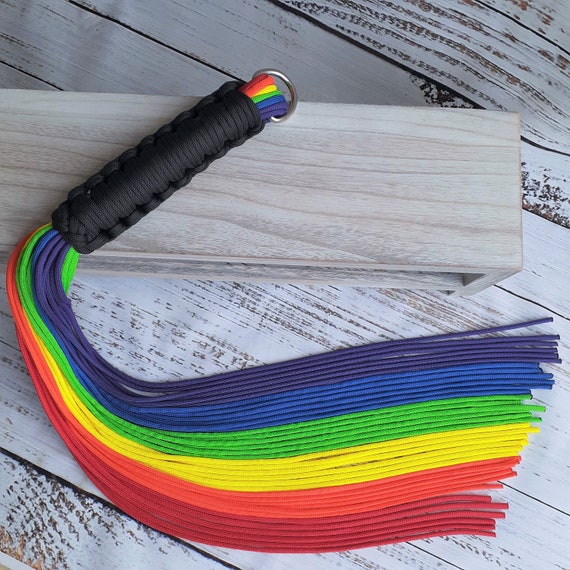The photograph features a whip with a handgrip style. The handle, located in the upper left corner of the image, is corded black. Attached to the handle are multi-colored tassels, grouped in distinct bands of dark blue, blue, green, yellow, red, and dark red, creating a vibrant rainbow effect reminiscent of LGBTQ pride symbolism. The tassels, likely made from soft cotton material, suggest a non-intimidating, potentially celebratory purpose. The whip rests upon a large white wooden table, which appears a bit worn with some visible paint chipping. Above the table is a smaller piece of white wood, further providing a layered backdrop to the scene. The overall setting is simple, yet detailed, emphasizing the colorful and symbolic nature of the whip.